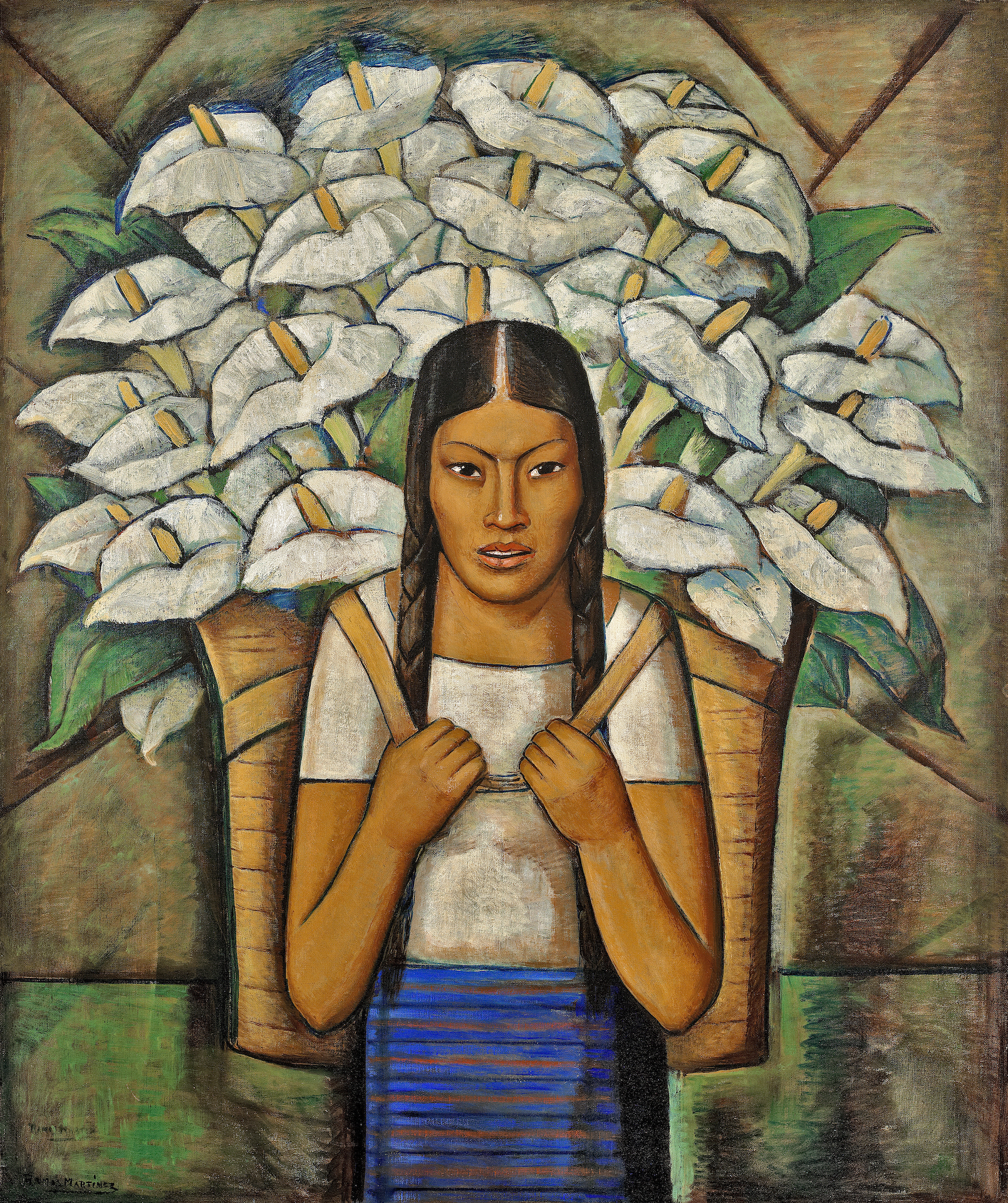This painting portrays a young woman with a dark olive or brown complexion and long dark hair, stylishly braided into pigtails on either side of her head, and parted in the middle. Her eyes are deep-set and dark brown, framed by a serious expression, while her thin lips show a hint of pink gloss. She wears a white short-sleeved t-shirt paired with a blue and brown striped skirt.

She carries a large straw basket on her back, filled to the brim with numerous white lilies, their light orange stems slightly visible. The basket, which is secured over her shoulders, is brimming with layers of these elegant flowers, giving a sense of their rich abundance.

In the background, a geometrically patterned wall in muted tans, greens, and browns enhances the overall composition. The wall's triangle shapes punctuate the serene yet determined presence of the woman, whose posture suggests a purposeful grip on the basket, as if the precious cargo of flowers is too valuable to risk dropping.